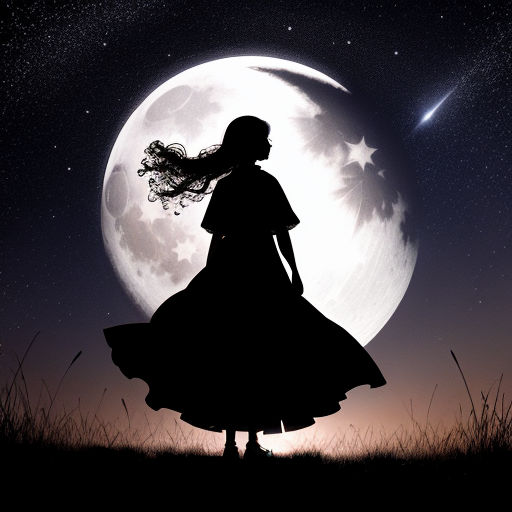In a stunning multi-color artistic piece set outdoors under natural night light, we see a vertically rectangular image featuring a central silhouette of a woman. She stands on a plot of tall grass, facing away from the viewer with her long hair beautifully flowing out behind her. Her dress, billowing as if caught in a gentle breeze, fans out around her, while her feet are adorned with discernible shoes. The backdrop is dominated by an enormous, glowing moon, larger than the silhouetted figure herself, with detailed gray craters. The night sky is a blend of deep blue, black, and soft brown hues dotted with twinkling stars. Towards the upper right corner, a bright shooting star appears to be on a collision course with the moon, creating a mesmerizing focal point in the serene, starry scene.